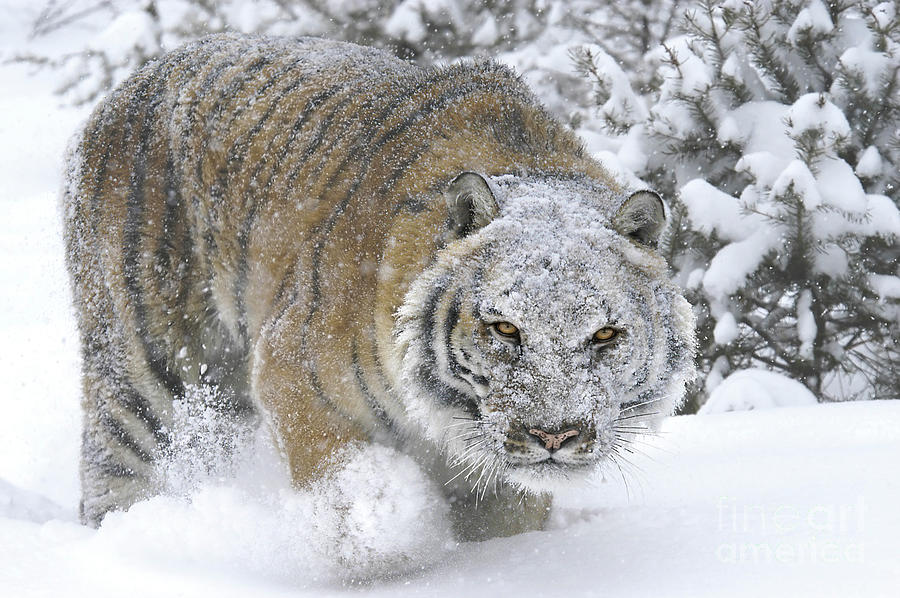A striking image captures a powerful tiger trekking through a snow-covered landscape. The tiger, adorned with classic orange and black stripes, has its face and whiskers dusted with snow and eyes that are a piercing orange hue, slightly different from the rest of its coat. Its pink nose stands out against the snowy backdrop. Snow clings to its body and legs, indicating that the snow is about a foot deep. In the background, the scene is filled with pine trees heavily laden with thick layers of snow on their branches, contributing to the wintry atmosphere. The tiger is moving towards the camera, kicking up snow with each step, and a sense of motion is conveyed by the snowflakes visibly falling around it. The photograph captures the raw beauty of the tiger against the stark white contrast of the snowy terrain during daytime.